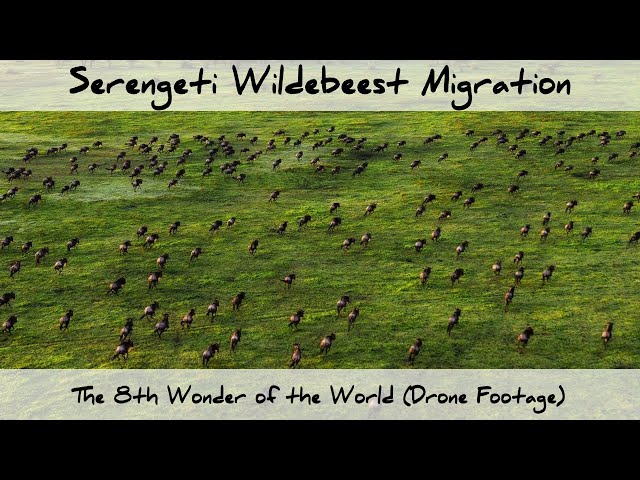This captivating image is a drone-captured screenshot titled "Serengeti Wildebeest Migration, the Eighth Wonder of the World," with the subtitle "drone footage" in parentheses at the bottom. The photograph showcases a sprawling, lush green field in the Serengeti, teeming with hundreds of wildebeest. These tan and black wildebeests appear in a dense, dynamic throng, all moving in the same direction across the vast pasture. The perspective is notably elevated, revealing the grandeur of this mass migration as the wildebeest stretch far into the distance, creating a mesmerizing visual of nature in motion. The image is framed with black borders at the top and bottom, and the text is displayed clearly in black with a white highlight, resembling a Youtube video thumbnail. This overhead action shot vividly captures the essence of this natural phenomenon, hailed as the Eighth Wonder of the World.